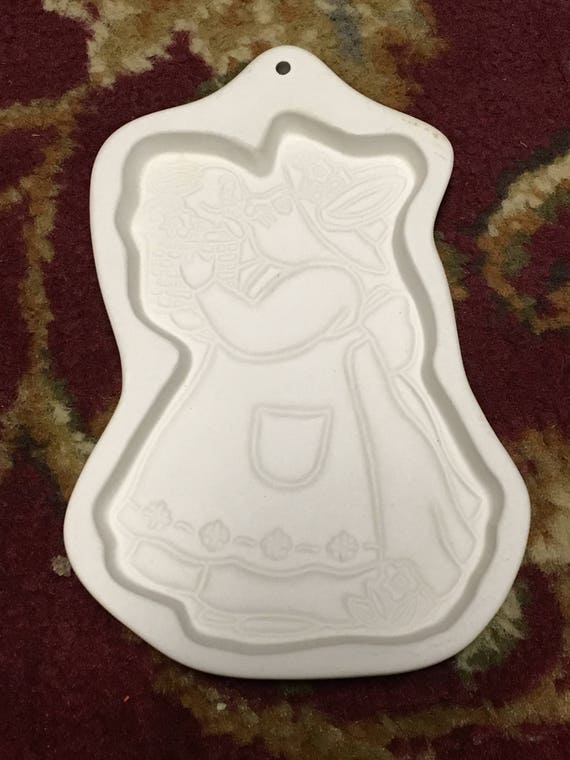The image showcases a detailed cake pan mold placed on a richly veined granite countertop, which features a striking brown hue with intricate veining. The cake pan, made from silver metal and designed for hanging with a small circle at the top, vividly depicts a bunny rabbit character facing left. The bunny, wearing a sun hat adorned with flowers, has elongated rabbit ears and a humanoid face. It dons an apron decorated with flowers and a pocket, along with a long skirt that flows down to its feet, also adorned with a flower. The front legs, resembling human arms, hold up a basket filled with flowers, completing this charming and elaborate design. The bottom surface of the pan is embossed with detailed impressions typical of a high-quality mold.